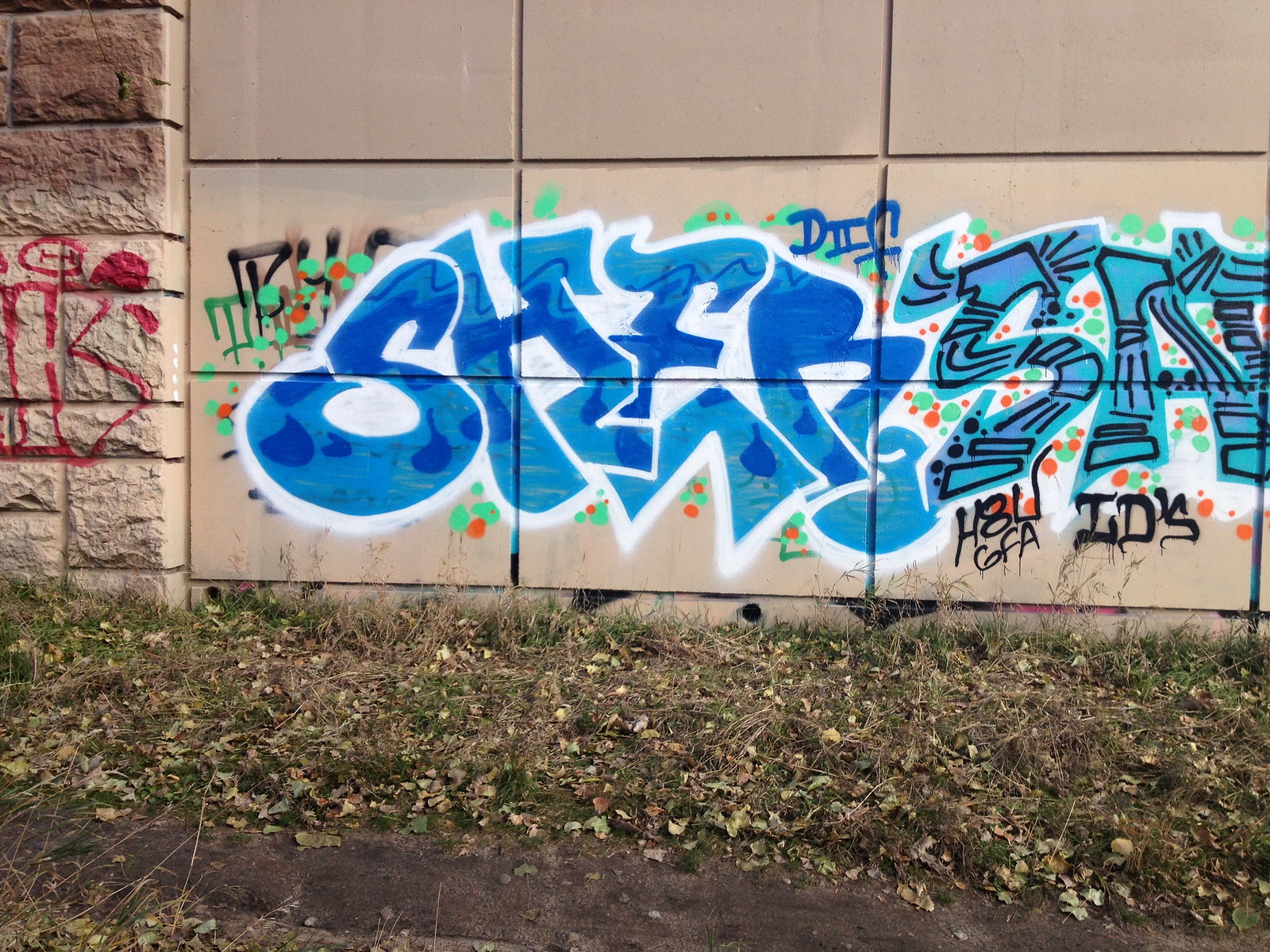The image depicts an outdoor scene featuring a pathway bordered by a mix of green and brown, overgrown grass alongside a building. The building itself is covered with off-white tiles, and adjacent to it is another structure made of smaller, rougher brown bricks. Dominating the visual are two walls; the first wall, constructed from light gray bricks, is adorned with intricate graffiti. The graffiti, predominately in shades of blue with black stripes, spells out the letters "S," "E," and "B," interspersed with red and green dots. In the bottom right corner of this wall, "ID's" is visible in black spray paint. The second wall to the left, composed of textured brown bricks, also features fragmented red graffiti that is difficult to decipher. The overall scene is one of urban decay and vibrant street art.